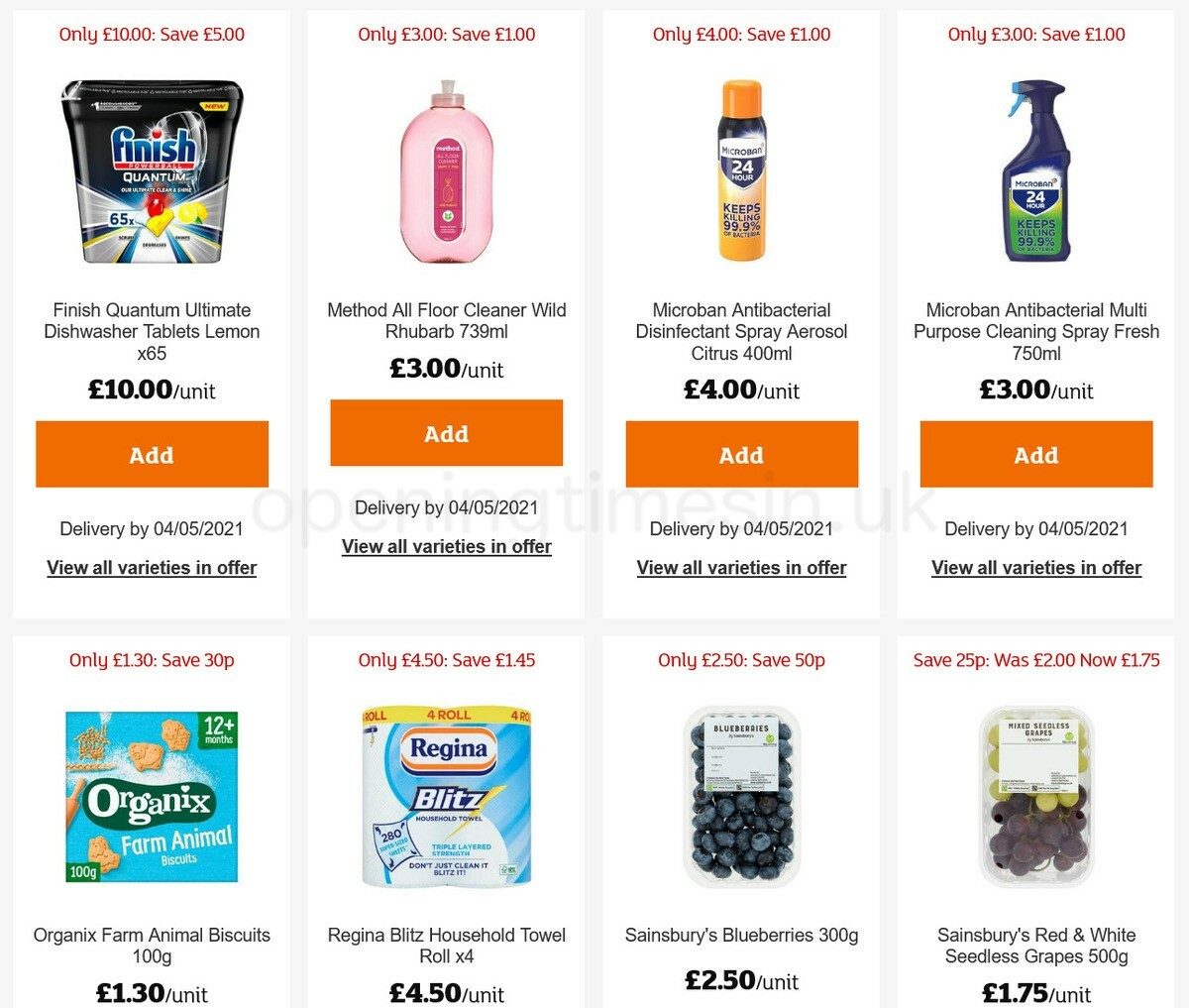The image displays various items available for purchase, set against a white background. Starting from the upper left-hand corner, the items are as follows:

1. **Finish Quantum Ultra Dishwasher Tablets** - Lemon scent, 65 tablets per pack, priced at £10 per unit. There's an orange "Add" button next to it and a note indicating delivery by 4th May 2021. Additional options and offers are available to view.

2. **Method All Floor Cleaner** - Wild Rhubarb scent, 739 milliliters, priced at £3 per unit. Includes an "Add" button and delivery by 4th May 2021. More varieties and offers can be viewed.

3. **Microban Antibacterial Disinfectant Spray Aerosol** - Citrus scent, 400 milliliters, priced at £4 per unit. Features an "Add" button and delivery by 4th May 2021.

4. **Microban Antibacterial Multipurpose Cleaning Spray** - Fresh scent, 750 milliliters, priced at £3 per unit, accompanied by another "Add" button.

At the bottom of the image, additional products are listed:

5. **Organic Farm Animal Biscuits** - 100 grams, priced at £130 per unit.
   
6. **Regina Blitz Household Towel Roll** - Priced at £450 per unit.

7. **Sainsbury’s Blueberries** - 300 grams, priced at £2.50 per unit.

8. **Sainsbury’s Red and White Seedless Grapes** - 500 grams, priced at £1.75 per unit.

Each product is accompanied by an image above its description, giving a visual representation of the items for sale.